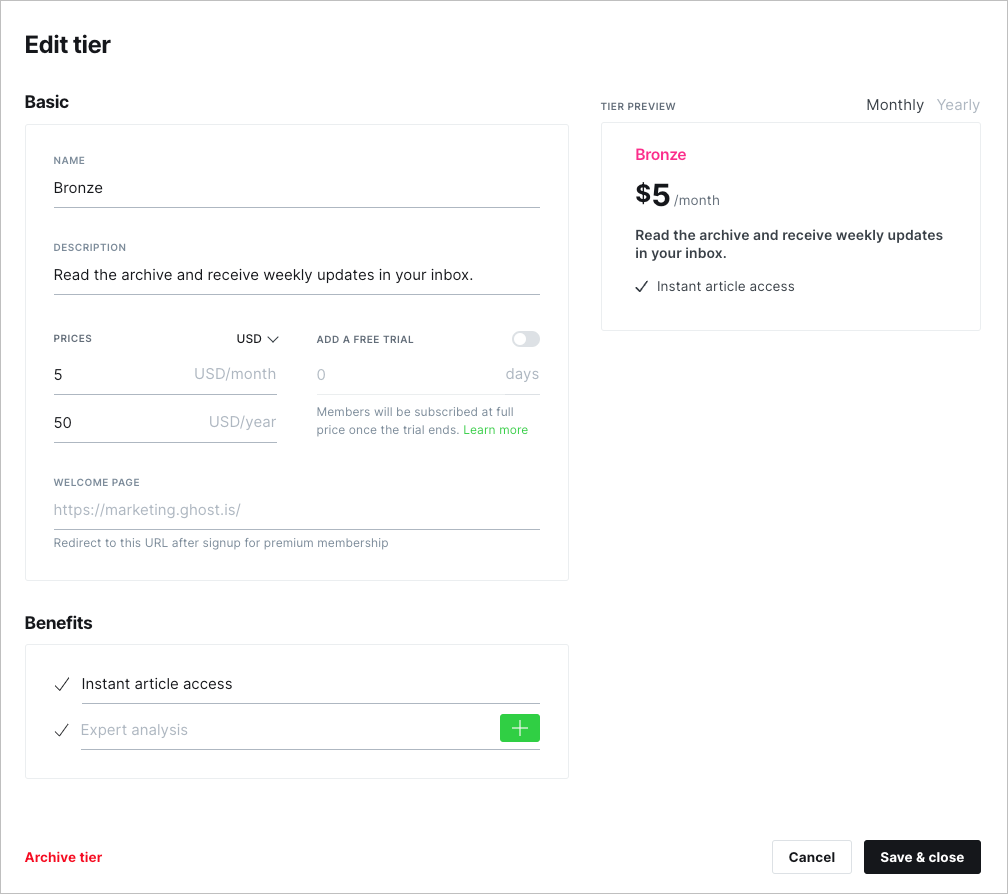This vertical image appears to be a screenshot taken from a smartphone or a webpage, viewed on a computer. The white background of the computer screen fills the entire backdrop, framed by a thin black line along all four edges. The top section prominently features bold black text. On the left side, it reads "Edit Tier," and in slightly smaller but still bold font, it says "Basic."

Below this, there is a box outlined in light gray with the following details:
- **Name:** Bronze
- **Description:** Read the archive and receive weekly updates in your inbox.
- **Price:** $5 USD per month, $50 USD per year.

Further along, there's a section labeled "Welcome Page" and a redirect URL option for premium membership sign-ups. There is an option to add a free trial, with the toggle currently set to off, indicating zero days. It mentions that members will be subscribed at full price once the trial ends. There is also a link to learn more.

Under the "Benefits" section, which is also in bold, it lists:
- Instant article access
- Expert analysis

A green plus sign button is shown, indicating the ability to archive the tier.

On the right-hand side of the image, there is a "Tier Preview" section. Users can toggle between monthly and yearly subscriptions, with the "Monthly" option highlighted. It indicates the Bronze tier is $5 USD per month. At the bottom, options to "Cancel" or "Save and Close" are displayed.